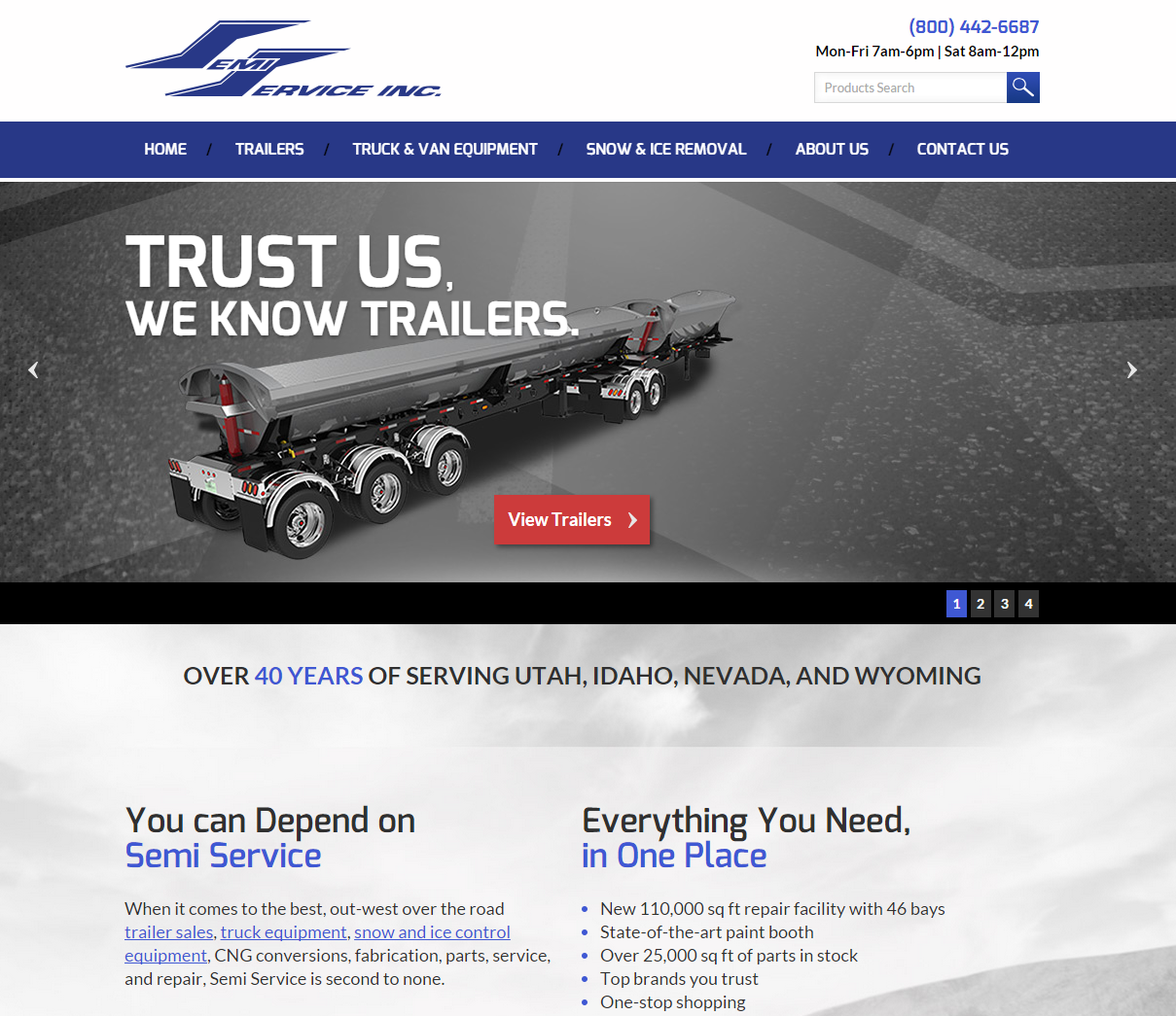This is a highly detailed screenshot of the SemiService.inc website, a tractor-trailer service company. On the upper right corner, set against a white background, the company’s logo and name are prominently displayed. The name "SemiService.inc" is written in blue, with the S's in "Semi" and "Service" stylized as angular S’s. Adjacent to this, also in blue, the company’s phone number (800-442-6687) is easily visible. Below the phone number, the operational hours in black text state: "Monday through Friday, 7 a.m. to 6 p.m.; Saturday, 8 a.m. to 12 p.m."

Directly beneath, a functional search bar accompanies a blue magnifying glass button. The placeholder text in the search bar reads "Products Search" in gray.

Following this is a blue navigation bar with white text, featuring menu options: Home, Trailers, Truck and Van Equipment, Snow and Ice Removal, About Us, and Contact Us.

Further down, against a gray background adorned with darker gray and white graphics, bold, all-capitalized white letters declare, "Trust Us, We Know Trailers." This is paired with an image of a semi-truck trailer, showcasing the portion that attaches to the truck and holds the load, complete with five sets of wheels. To the right of this image, a vivid red button with white text offers a clear call to action: "View Trailers."